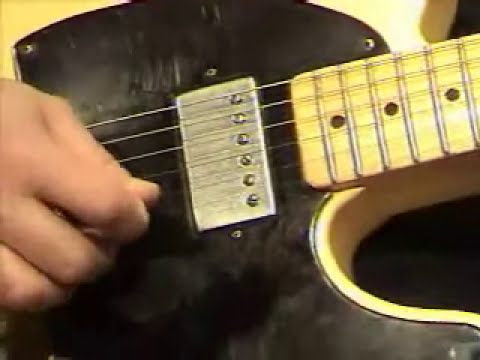This detailed close-up shows a guitarist's hand poised to strum an electric guitar. The guitar predominantly features black and yellow hues, or possibly a hollow body design with light wood tones. Visible on the body are signs of wear, like fingerprints and marks, hinting at extensive use. Integral components include the metallic pickups with six screws, adding a silvery contrast to the black plate beneath the strings. The neck of the guitar showcases a light brown wooden color, adorned with silver frets and black dot inlays. The background is a stark black, drawing focus to the intricate details of the instrument and the hand, possibly Caucasian, preparing to play the strings.